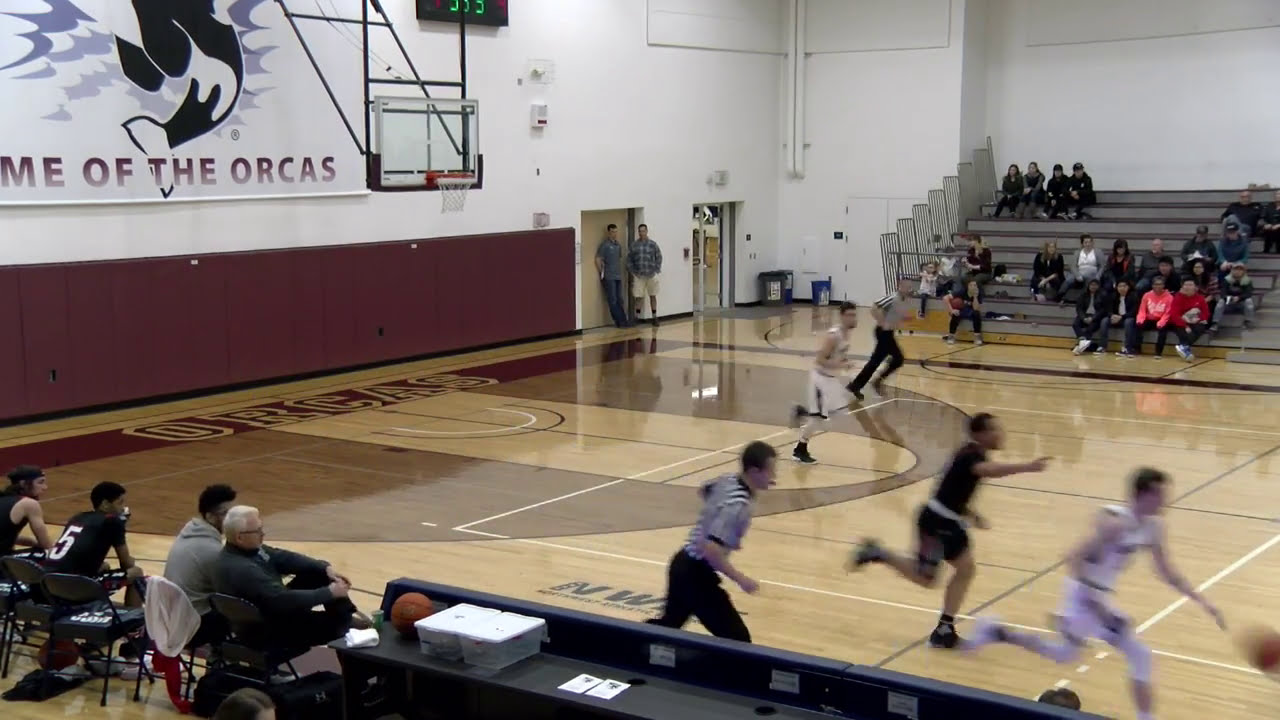The image depicts a high school basketball game taking place in an indoor gymnasium. The gym's floor is made of light-colored, polished wood, and the walls are painted white. The home team's side of the court is marked by a "Home of the Orcas" sign in a darker red background with the team's name in a varsity-style font. There is a basketball hoop and backboard on the left wall, where a player dressed in white is holding the ball, moving towards the right side of the image, followed by other players dressed in either white or black uniforms, as well as a referee. The scene is dynamic, with several players running across the court. Spectators are seated on bleachers positioned on the upper right side of the image and two individuals can be seen leaning against the wall near a door in the middle top section. At the bottom middle, near the edge of the image, there is a scorekeeper's desk and on the lower left corner, players and a coach are seated on folding chairs. The image captures the intense moment of the game in a vividly bustling gym environment.